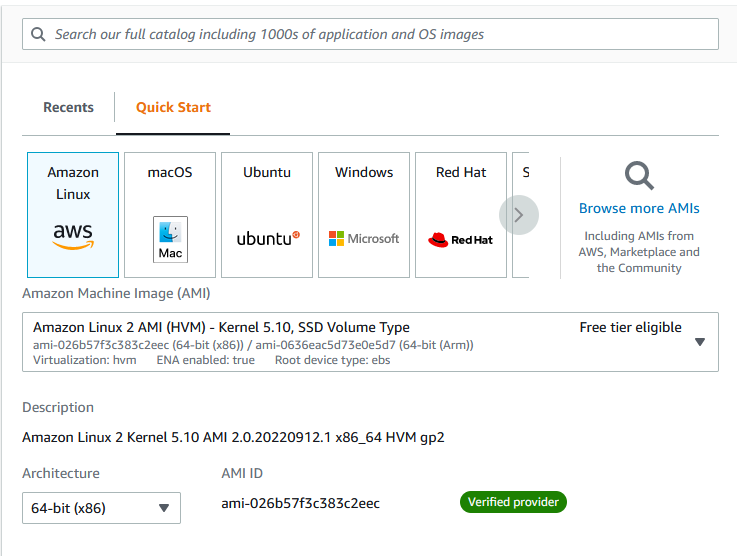Detailed Caption:

This screenshot captures a webpage dedicated to Amazon marketing. At the top, there's a prominent search window featuring a magnifying glass icon where users can input data. The placeholder text within the search bar reads, "Search our full catalog including thousands of applications or application and OS images" in gray text.

Immediately below the search bar, a white background displays text in both gray and orange fonts. The gray text reads "Recents" while the orange text, situated to the right separated by a vertical dividing line and left-justified, reads "Quick Start."

Further down, another dividing line separates a series of square options representing different operating systems, each accompanied by their respective logos. The options visible are:
- Amazon Linux, with the AWS logo
- macOS, with the macOS logo
- Ubuntu, with its logo
- Windows, with the Microsoft logo
- Red Hat, with the Red Hat logo

Additional options are present but not visible in this part of the interface. Below these options, a magnifying glass icon and blue text prompt users to "Browse more AMIs."

Underneath this section, detailed technical information about an Amazon Machine Image (AMI) is provided:
- AMI: Amazon Linux
- Kernel: 5.10
- Volume type: SSD
- Technical details, including a description and location within the interface
- Architecture: 64-bit
- AMI ID

In the bottom right corner of the screenshot, a green toggle button with white text indicates "Verified Provider."